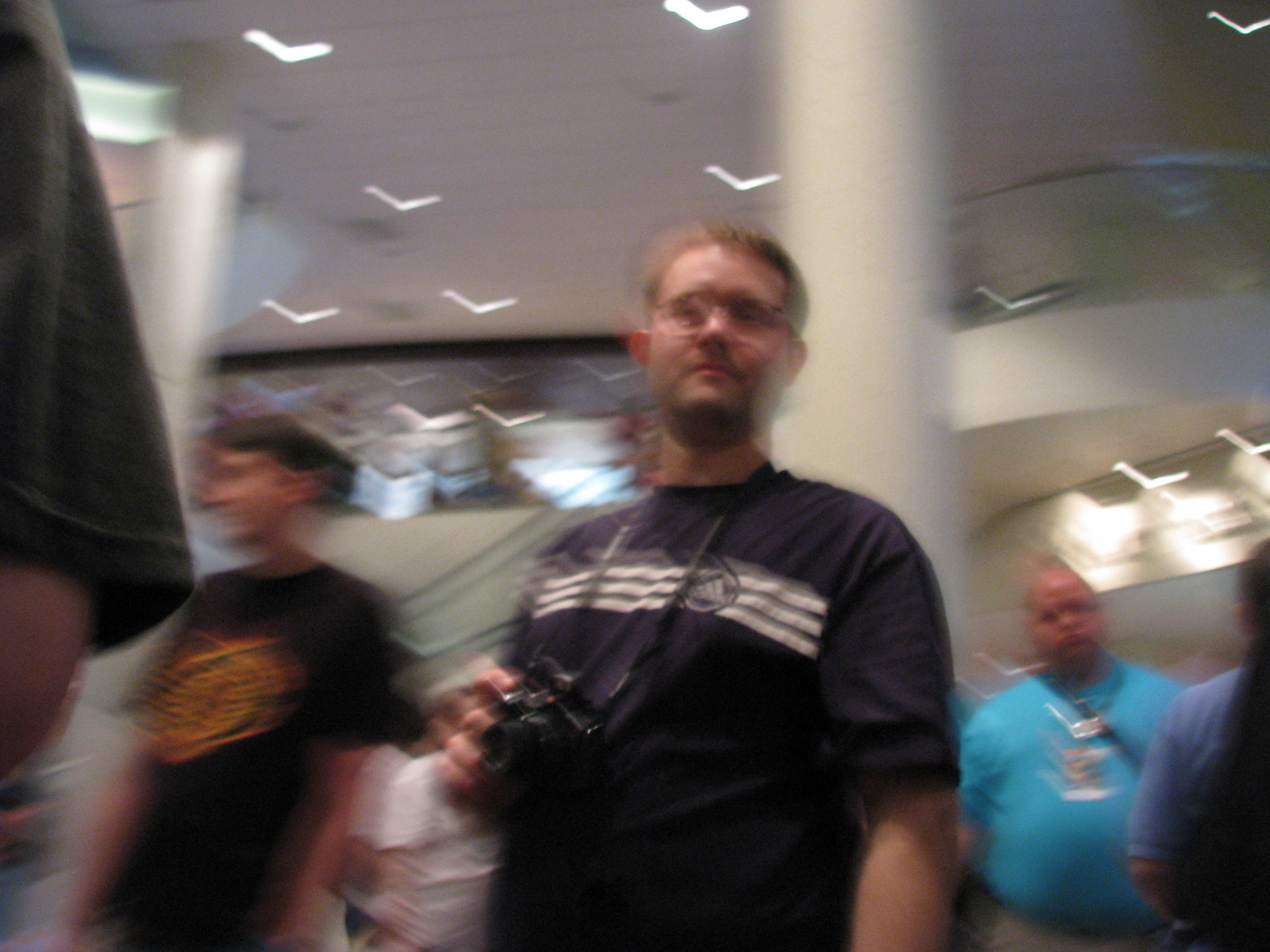In this slightly blurry photograph, a group of people gather at what appears to be a convention or meeting, possibly held in a multi-level venue. The background reveals an upstairs area with white columns and railings, adding a sense of architectural elegance. At the center of the image stands a man dressed in a dark-colored Adidas t-shirt, distinguished by white stripes across the chest. He holds a small camera dangling from his neck with one hand, indicating an interest in photography or documentation. The man is white, has short hair, wears glasses, and sports a neat, short facial hair. Flanking him are two other individuals; one on the right clothed in a blue shirt, and one on the left donning a dark brownish shirt. The overall blurriness of the image suggests that the camera was in motion as the picture was taken, leading to an out-of-focus effect.